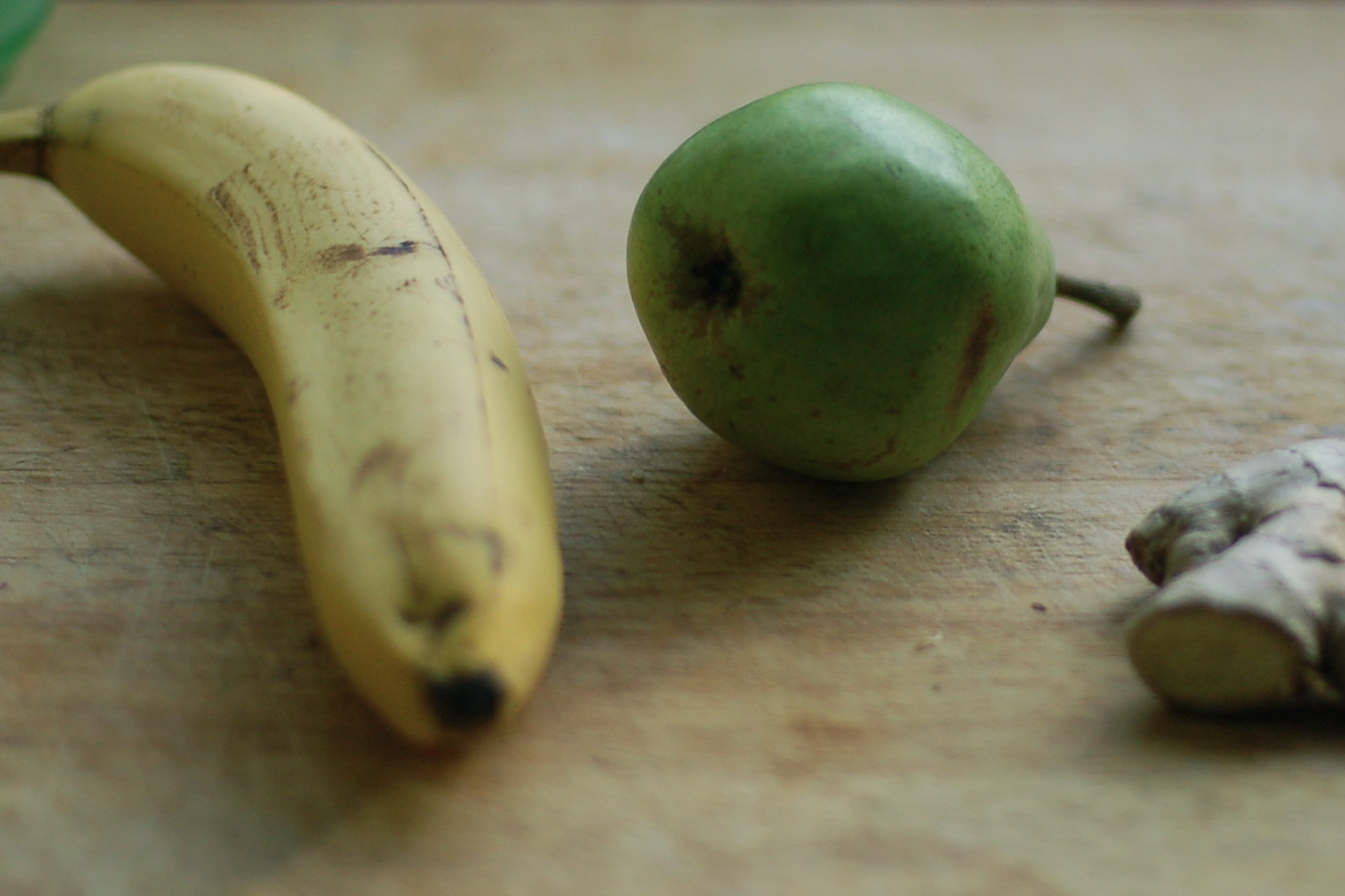This high-quality photograph, taken with an advanced camera, captures a detailed still life composition on an unpainted wooden table. In the foreground, three distinct objects are arranged meticulously – a ripe banana, a green pear, and what appears to be a piece of ginger root.

On the left, the banana lies mostly in view with its stem slightly off the image. The fruit showcases a few black spots, indicating its ripe and ready-to-eat stage. Positioned centrally, the green pear stands upright, displaying slight blemishes and brown marks around its stem and sides, suggestive of its freshness. To the right, a piece of ginger root, partially cut and soft in appearance, extends out of the frame, offering a hint of its gnarled texture.

The photograph employs a shallow depth of field, blurring the wooden table's background while keeping the textures and ridges of the unpainted wood subtly visible. The blurred background enhances the clarity and focus on the three objects, creating a striking contrast. This well-composed image effectively uses focus and perspective to draw attention to the natural qualities and details of the still life subjects.